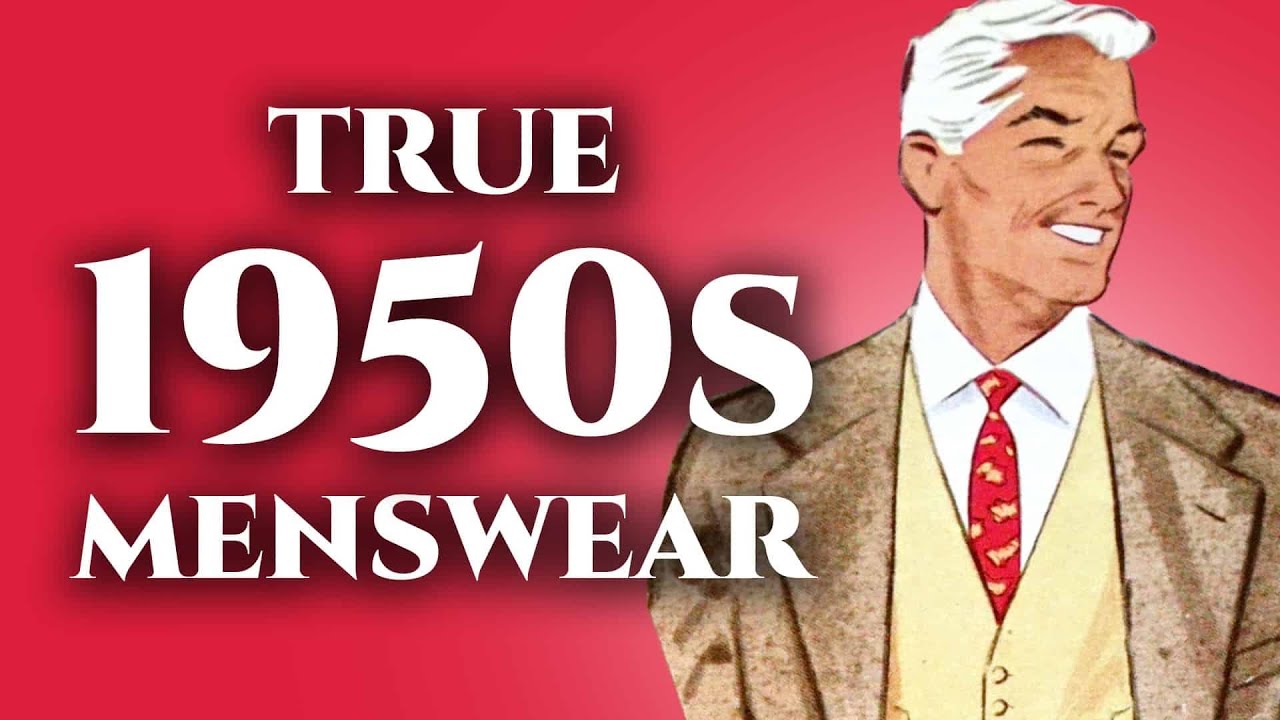The image features an illustrated older gentleman, depicted with short white hair and bushy eyebrows, smiling broadly to his left. His eyes are partially closed, adding to his cheerful demeanor. He sports a traditional 1950s-style brown suit, complemented by a yellow undercoat and a crisp white shirt. The red tie he is wearing appears to have a leaf pattern, potentially maple leaves. The background is a red gradient, becoming whiter behind the man, giving it a retro aesthetic. On the left side, the text "True 1950s Menswear" is prominently displayed in white print with a slight shadow effect, suggesting a vintage advertisement. The entire composition merges hand-drawn illustration with computer-generated elements, evoking a nostalgic tribute to mid-20th century men's fashion, reminiscent of the 'Mad Men' era.